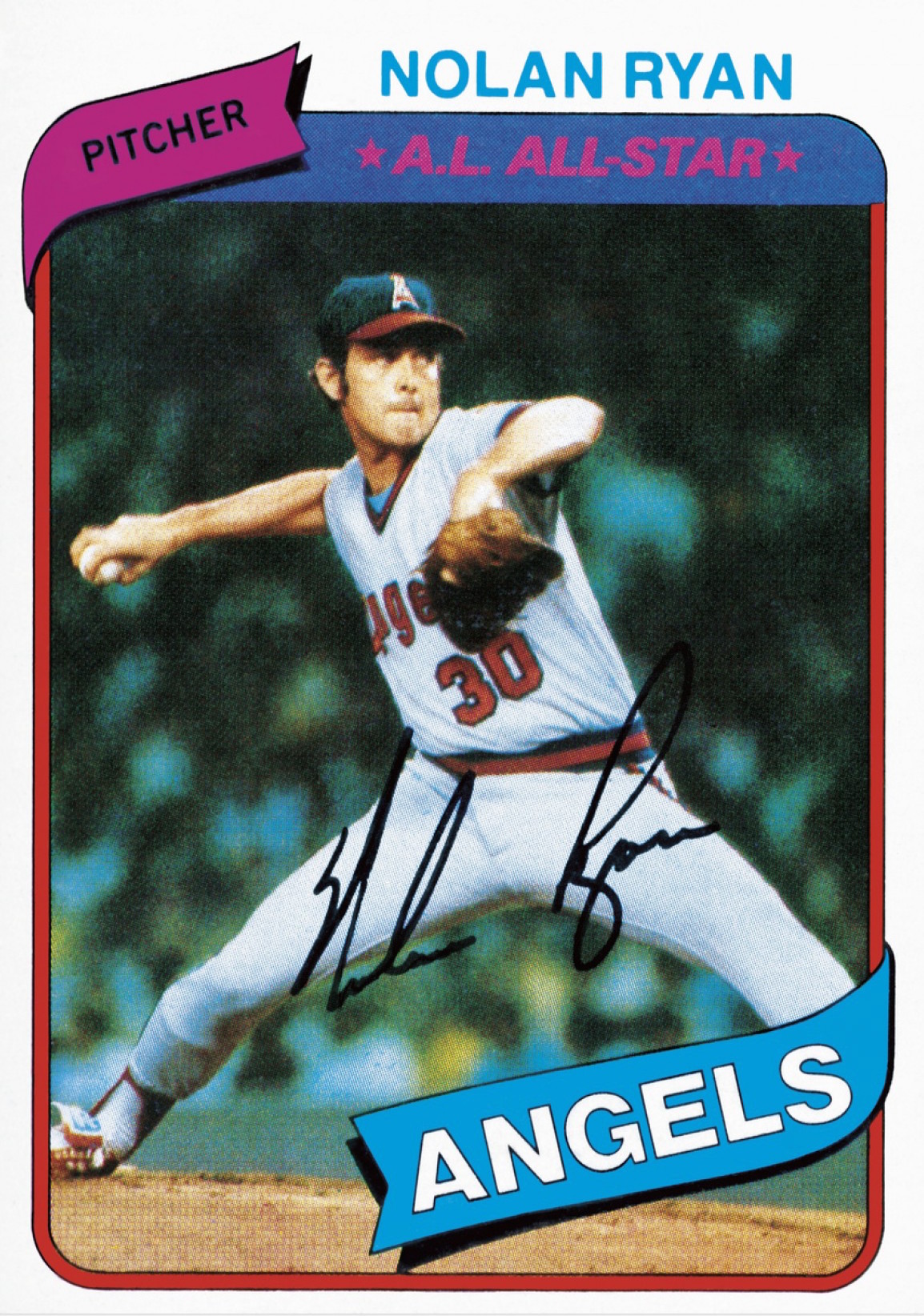This rectangular, vertical poster features baseball legend Nolan Ryan, prominently positioned in the center wearing his white uniform emblazoned with the number 30. Ryan is captured mid-pitch, his intense focus evident as he grips the baseball in his right hand and wears a baseball glove on his left. He sports a navy blue cap with a red brim, marked with a red 'A', signifying his team, the Angels. His signature is elegantly scripted across the front of the poster in black ink. The top of the poster boasts "All Star, A.L. All Star" in bold red letters, while a purple banner with black letters is present in the upper left-hand corner. The bottom of the poster highlights "Angels" in white letters against a blue background ribbon. Additionally, "Nolan Ryan" is displayed in blue at the top, framed by the overall red border of the card, marking it as a collectible baseball card.